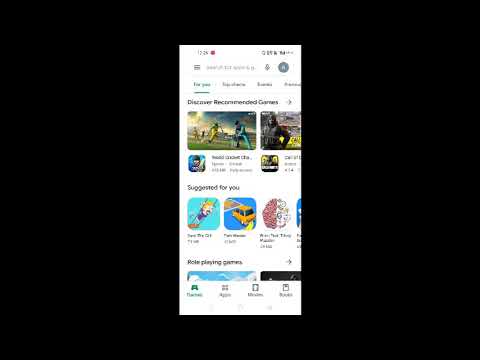This image is a detailed screenshot of a mobile phone displaying an app store interface, set against a black background. The phone is centered within the image, and the app store screen has a predominantly white backdrop. Although the time displayed on the phone is blurry, it appears to be either 2:25 or 12:25. 

At the top of the screen, there's a search bar and a user icon. The interface includes several navigational tabs, such as "For You." Featured content in the app store is organized under various headings and thumbnails showcasing different games. The first heading, "Discover Recommended Games," displays a partial view of two game options through one and a half screenshots. 

The next section, "Suggested for You," highlights three distinct game suggestions: the first appears to be a children's game featuring an image of a child on a swing; the second resembles a parking game with a car depicted on a blue field; and the third seems to be a brain teaser, indicated by the illustration of a brain.

The last visible section is labeled "Role-Playing Games," although no specific games from this category are detailed in the description. Each segment is visually segregated, making it easy to differentiate between the types of games being recommended.